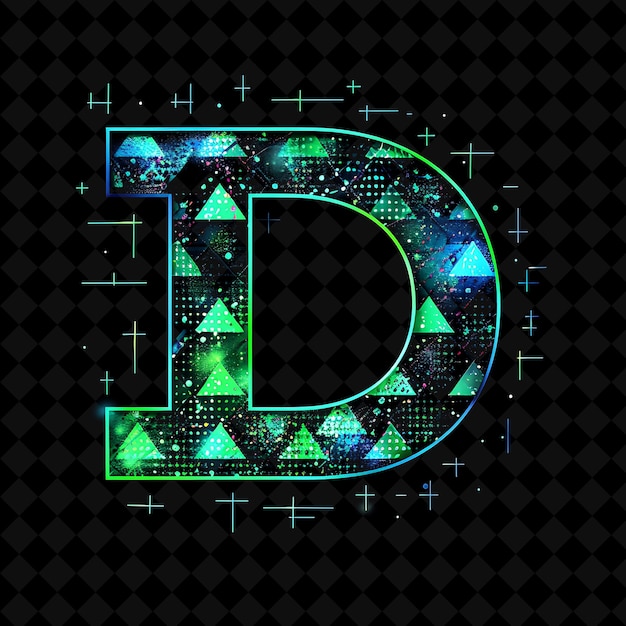The image features a striking, large capital letter "D" set against a backdrop of alternating dark gray and medium gray diamond patterns. These diamond shapes, which are essentially squares turned on their sides, cover the entire background horizontally. The "D" itself is outlined with a gradient that shifts between vibrant shades of blue and green, creating an eye-catching neon effect.

Inside the "D" are numerous equilateral triangles of varying shades of green and blue, some with gradient fills. These triangles are strategically placed to create a pattern within the "D," contrasting against its black hollow center. Surrounding the letter, there are various smaller dots and circles in multiple sizes, adding complexity and depth to the design.

Additionally, there are intricate crisscross patterns, vertical and horizontal lines, and forms resembling crosses and H shapes that further embellish the area around the "D." These lines and shapes range in color, primarily green, with variations in lightness and darkness as they extend outward. Some lines look like dashes or partial shapes, contributing to the layered, textured look.

Overall, the graphic design is rich with detail, featuring a play of light, color gradients, and geometric patterns that give it a dynamic, almost galaxy-inspired aesthetic.